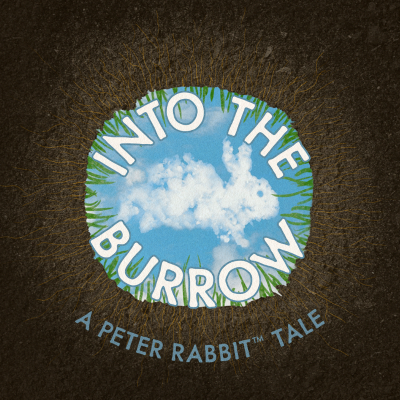The image is a cover scan of a book titled "Into the Burrow: A Peter Rabbit Tale." The centerpiece of the cover features a circular cut-out that reveals a clear blue sky with a fluffy white cloud shaped like a running rabbit, its ears pointed upward, evoking a sense of determination. Surrounding the sky and cloud are green blades of grass protruding upwards from the edges of the circular cut-out, simulating the view as if one were looking up from within a burrow. The outer texture of this viewing hole resembles dirt and intertwined roots. Encircling the top of the hole, the title "Into the Burrow" is written in white, with a blue outline, while the bottom displays "A Peter Rabbit Tale" in blue text. The overall design effectively immerses the viewer in the perspective of being inside a rabbit's burrow, gazing up at the open sky above.